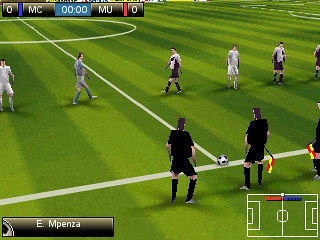This image appears to be a screenshot from a video game featuring a sports field. The field is characterized by a vividly green surface with distinct white markings delineating the boundaries and other key areas. The characters on the field are digitally rendered, resembling cartoon-like figures rather than real-life humans, suggesting a stylized aesthetic common in video games.

In the background, there are signs displaying the text "0MC0000MU0," which could be an in-game code or a stylized graphic element. Prominently in the foreground, a black banner bears the name "E. IMPENZA." Additionally, in the lower right corner of the image, there is a white inset diagram of the field, featuring white borders, goals on both ends, and a central mark indicating the middle of the field, providing a miniaturized overview of the playing area.